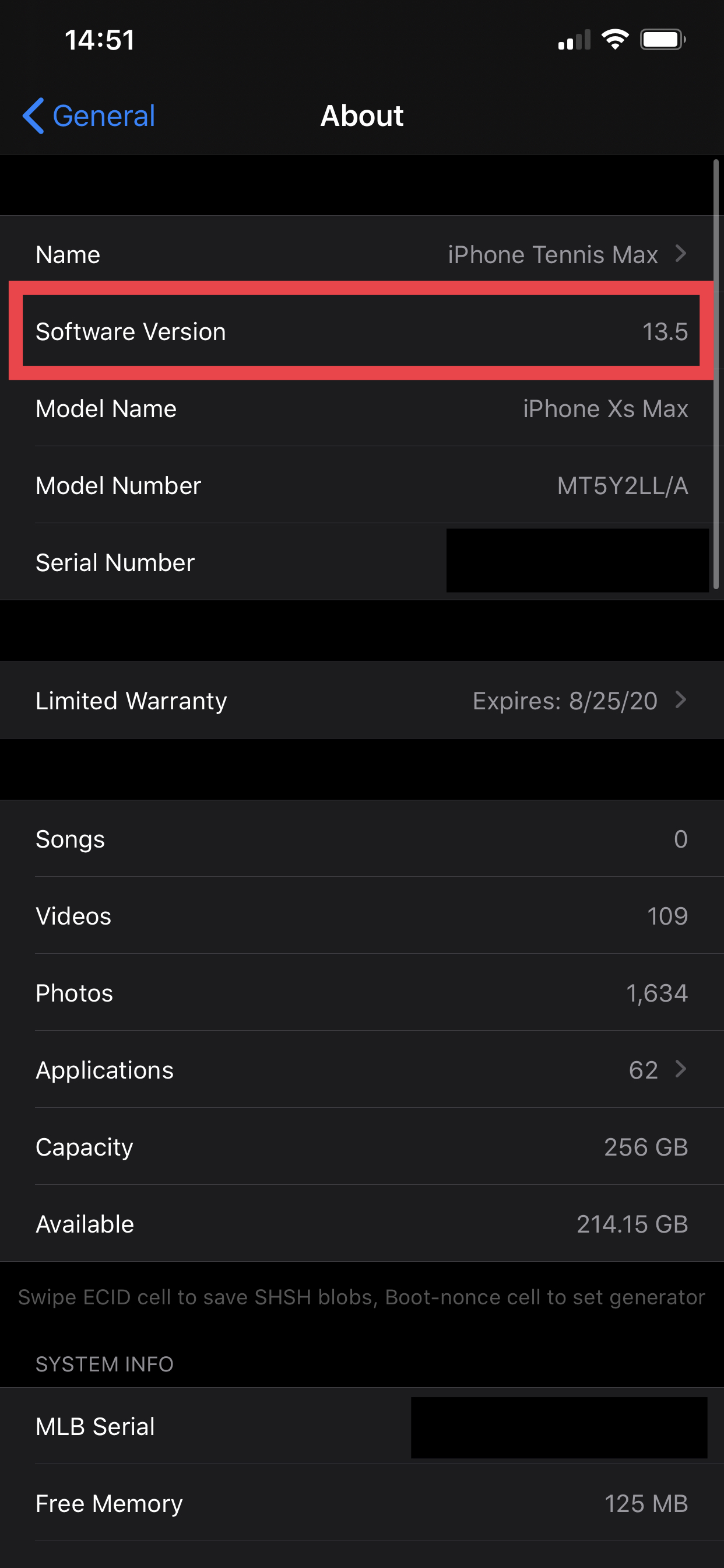The image depicts the 'About' section within the General Settings of an iPhone XS Max. The most prominent feature is a red box highlighting the text "Software Version 13.5" at the top right corner. The display reveals various details about the device, including the model name "iPhone XS Max," which is written in white text against a black background. Below this, other information such as the model number, serial number, and the status of the limited warranty, which expired in 2020, is listed. The section further includes counts of the songs, videos, photos, and apps stored on the device, as well as its capacity and available storage.

Additional visual elements include an arrow in the top left corner, also in white, indicating the option to go back to the General settings menu. The device time is shown in military format, 14:51, and the status bar at the top right reveals the device has two bars of cellular service, Wi-Fi connectivity, and a fully charged battery. The use of military time suggests that the iPhone user might be outside the United States.